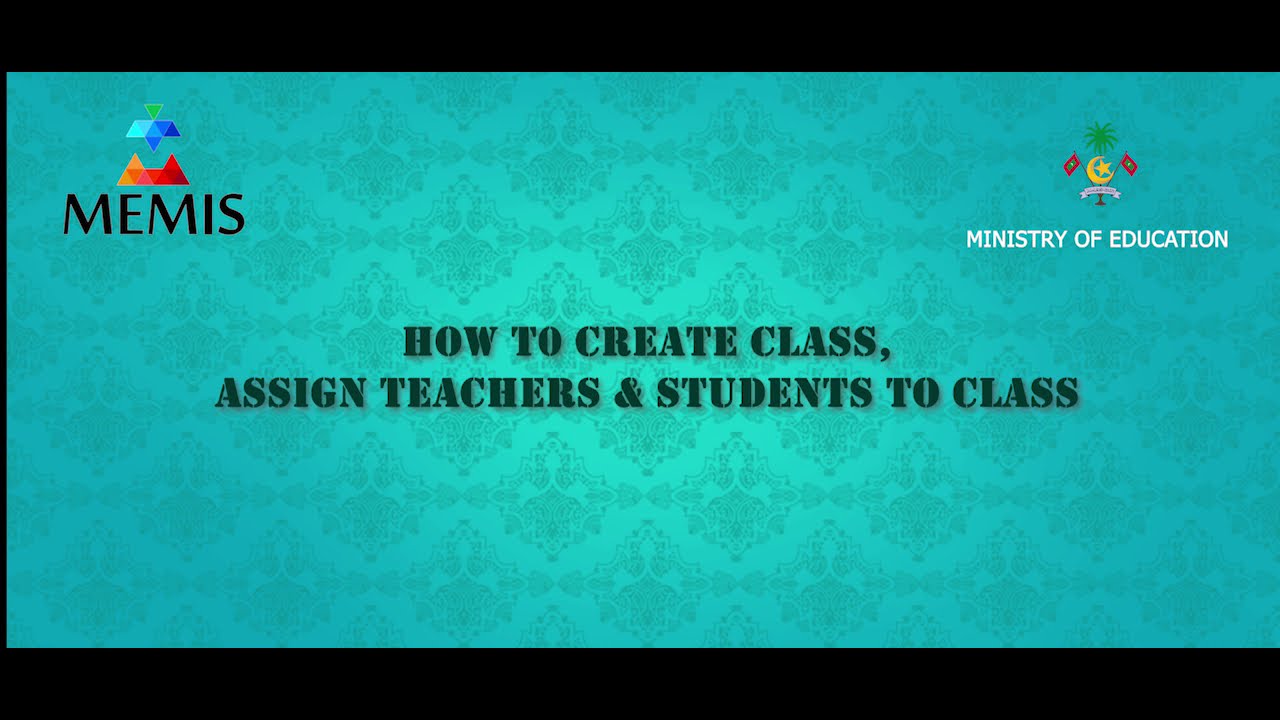This image appears to be the introduction slide to a presentation, characterized by an ornate bluish-green background that features a subtle, decorative pattern reminiscent of wallpaper. The background color gradient is lighter at the center and darkens towards the edges. Along the top and bottom of the image are modest black borders framing the primary content.

In the upper left corner, there is a logo consisting of geometric shapes, with the text "M-E-M-I-S" in bold, black capital letters beneath it. On the upper right side, there is a more intricate logo, featuring a tree, flags, and what resembles a coat of arms, which identifies it as the emblem of the Ministry of Education of the Republic of Maldives, with this title written in clean white lettering below the logo.

Dominating the center of the slide is the main instructional text in black, printed in a large, serif stencil font that reads: "HOW TO CREATE CLASS," followed by a line break, and then "ASSIGN TEACHERS AND STUDENTS TO CLASS." The design and placement of the text suggest a clear emphasis, ensuring it captures the viewer's attention immediately. The overall color palette includes hues of teal, sea green, blue, alongside the black and white text and logos, set against the patterned backdrop, creating a sophisticated and informative presentation slide.